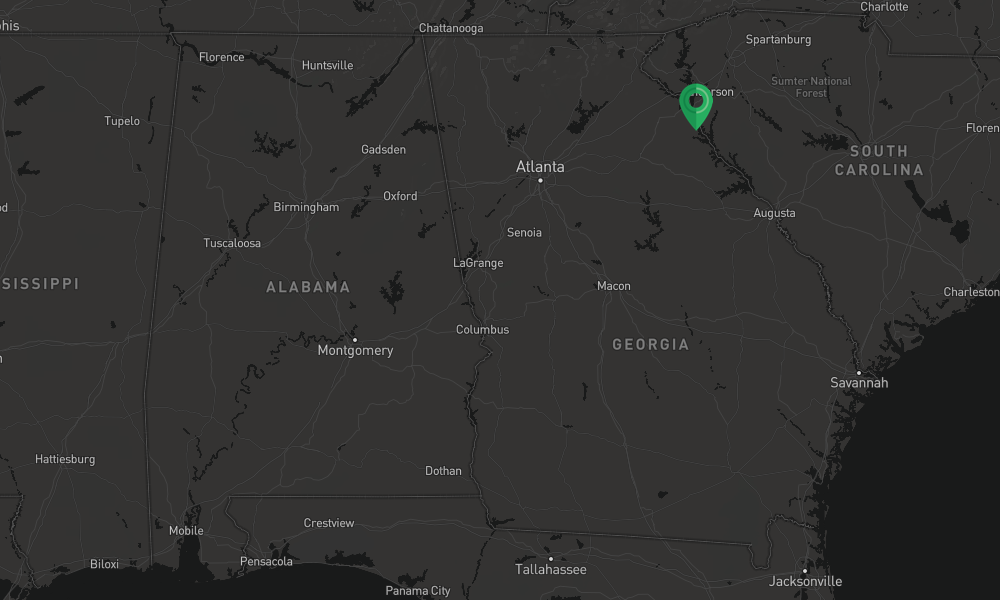This image features a detailed screenshot of a map, displayed in landscape mode, with a dark background. The focal point is a bright green location dot situated in the upper right section of the image, partially obscuring the letters "RSON." Directly southeast of this marker, a highway or significant road leads us to Augusta, pinpointing the setting as likely being Augusta, Georgia.

In the upper left-hand corner, the letters "HIS" are visible. The map spans horizontally to include Chattanooga in Tennessee, followed by Spartanburg, and further east we find Charlotte in the upper right-hand corner. The same region highlights Sumter National Forest within South Carolina, aptly labeled in capital letters.

Descending the right side of the map, we spot Florence followed by Charleston. Transitioning to the left side of the image, notable locations include Tupelo, Mississippi, then Hattiesburg, and Biloxi. At the bottom edge of the map, stretching from left to right, the cities listed are Biloxi, Mobile, Pensacola, Crestview, Panama City, Tallahassee, and Jacksonville, denoting the state of Florida.

Centrally positioned on the map are various cities spread across Alabama and Georgia, completing the detailed geographical representation.